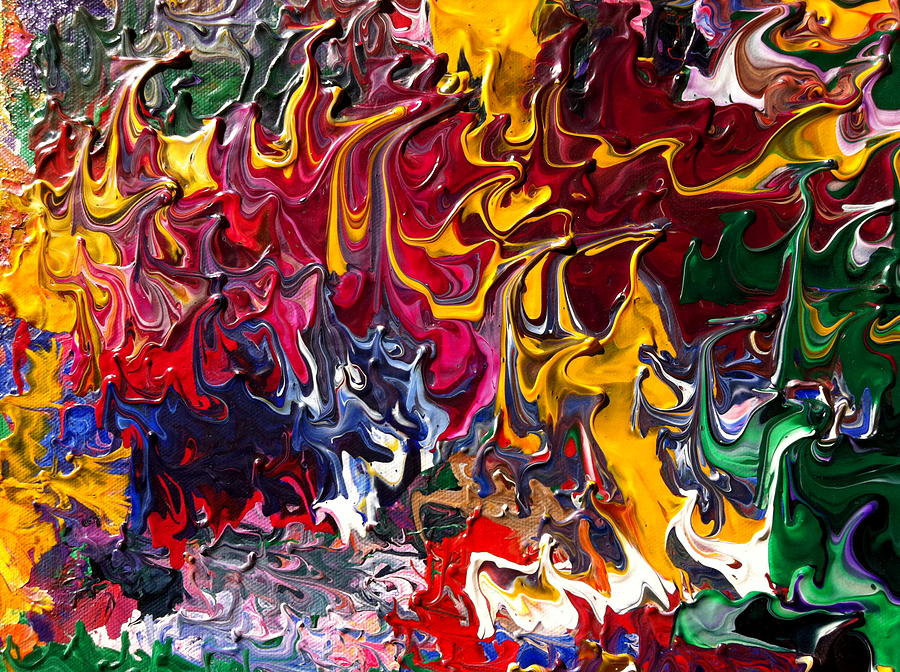This abstract painting is a vibrant explosion of color and texture, created using thick layers of acrylic or oil paint. The left side of the artwork predominantly features a blend of yellow and orange hues, mingling with reds towards the center. The bottom right of the painting showcases a mix of green and purple, while the top right transitions into a darker red. The very bottom, particularly on the left, highlights a white base with splashes of blue and red. The colors in the painting do not form solid fields but rather swirl and blend together in an almost wave-like pattern, creating an uneven yet intertwined effect. The heavy layering of the paint gives the piece a highly textural, tactile quality, making it appear rough, bumpy, and fiery as the paint moves upwards into dynamic points. The overall composition is bright and clear, with no discernible objects or figures, focusing purely on the interplay of color and form.